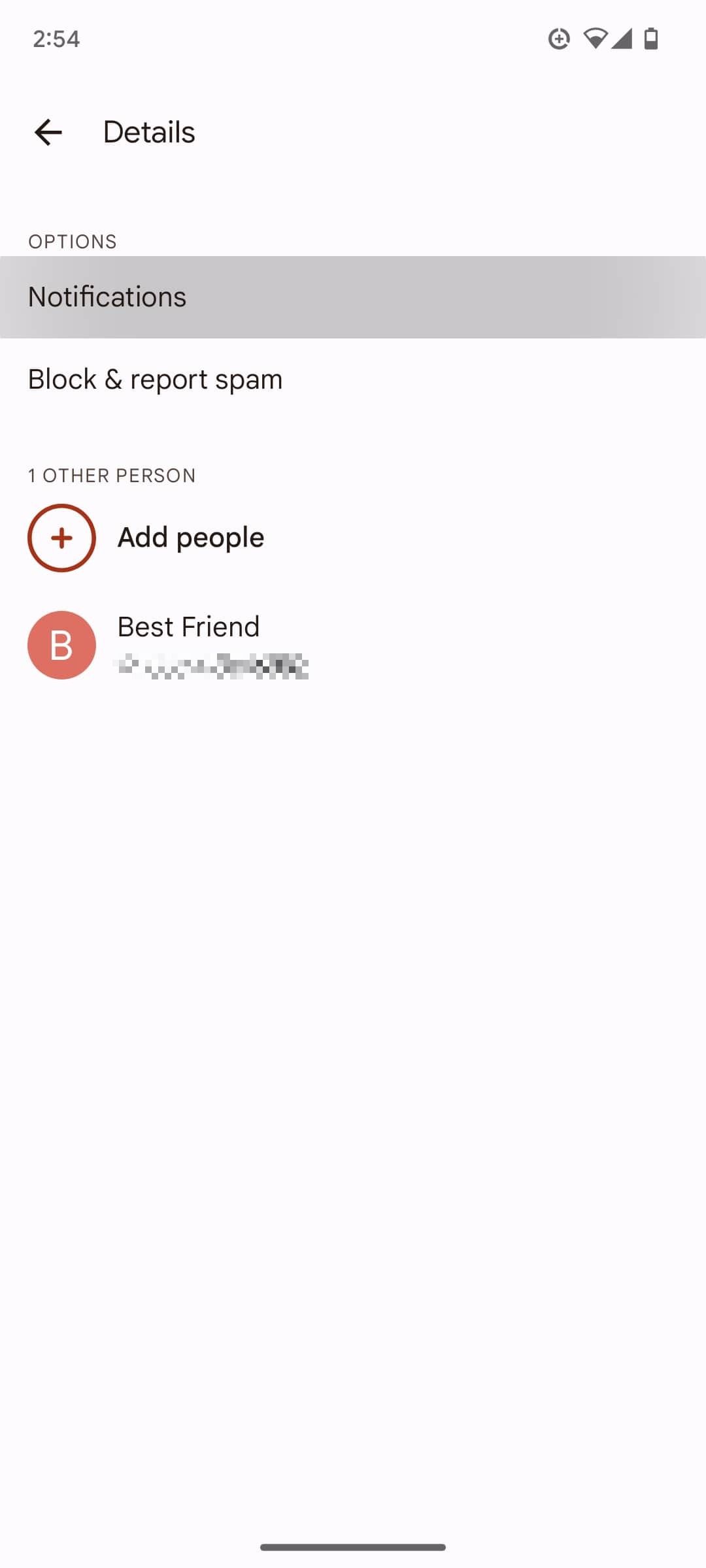This image showcases a smartphone screen displaying a website interface. The phone has a moderate signal strength and a battery level at approximately 50%. The time displayed in the top-left corner reads 2:54. Directly below the time, there is a back arrow labeled "Details." Beneath this, a gray bar features the word "Options" written across it.

Below the gray bar, the label "Notifications" appears, followed by two options: "Block" and "Report Spam." There is a small gap before the next section, which shows a red circle with a plus sign to the left of the text "Add People." Further down, there is an icon consisting of a white letter "B" set against an orange-red background, next to the words "Best Friend." The text underneath this segment is blurred and unreadable.

The lower portion of the interface is predominantly light gray, extending to the bottom of the screen. Concluding the view is a horizontal gray line across the very bottom of the page, indicating the simplistic nature of the site's design. The purpose or specific content of the page remains unidentified from the provided elements.